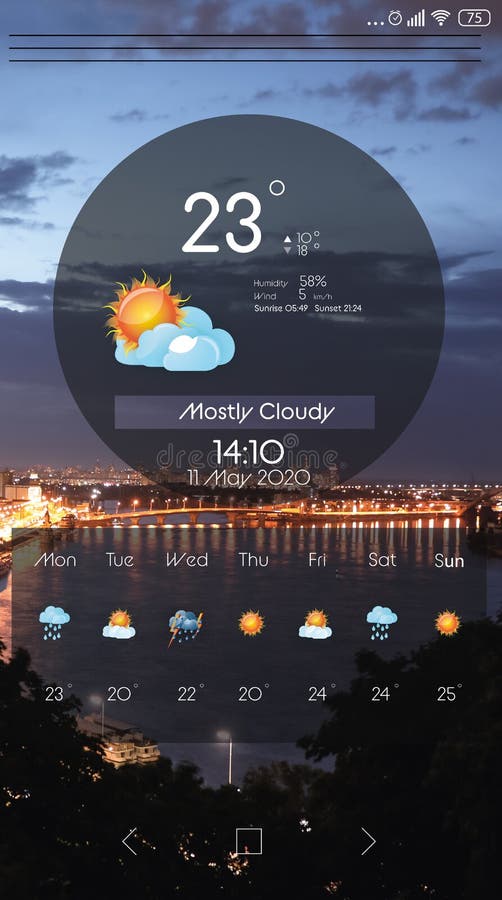This image is a detailed screenshot from a smartphone, showcasing a weather forecast application. In the upper right-hand corner of the screen, the battery icon indicates a charge level of 75%, alongside icons for Wi-Fi, wireless connection, and an alarm clock. 

The image depicts the weather forecast interface set against a scenic nighttime city backdrop featuring a prominent bridge over a river, although the specific city is unidentified. The sky is transitioning into nightfall with visible clouds darkening gradually.

Centered prominently at the top is a gray circular overlay displaying critical weather information. Within the circle, the temperature is shown as 23°C in white text. A stylized graphic of clouds and a yellow-orange sun accompanies the temperature, with the text "Mostly Cloudy" underneath. The precise time, "14:10," and the date, "11 May 2020," follow, providing further context.

Below this main section, a weekly weather forecast is presented in a row, listing the days from Monday to Sunday. Each day is accompanied by small icons depicting various weather conditions, such as rain or sun, along with the corresponding temperatures for each day.

Overall, the screenshot offers a comprehensive and visually appealing summary of the current and upcoming weather conditions.